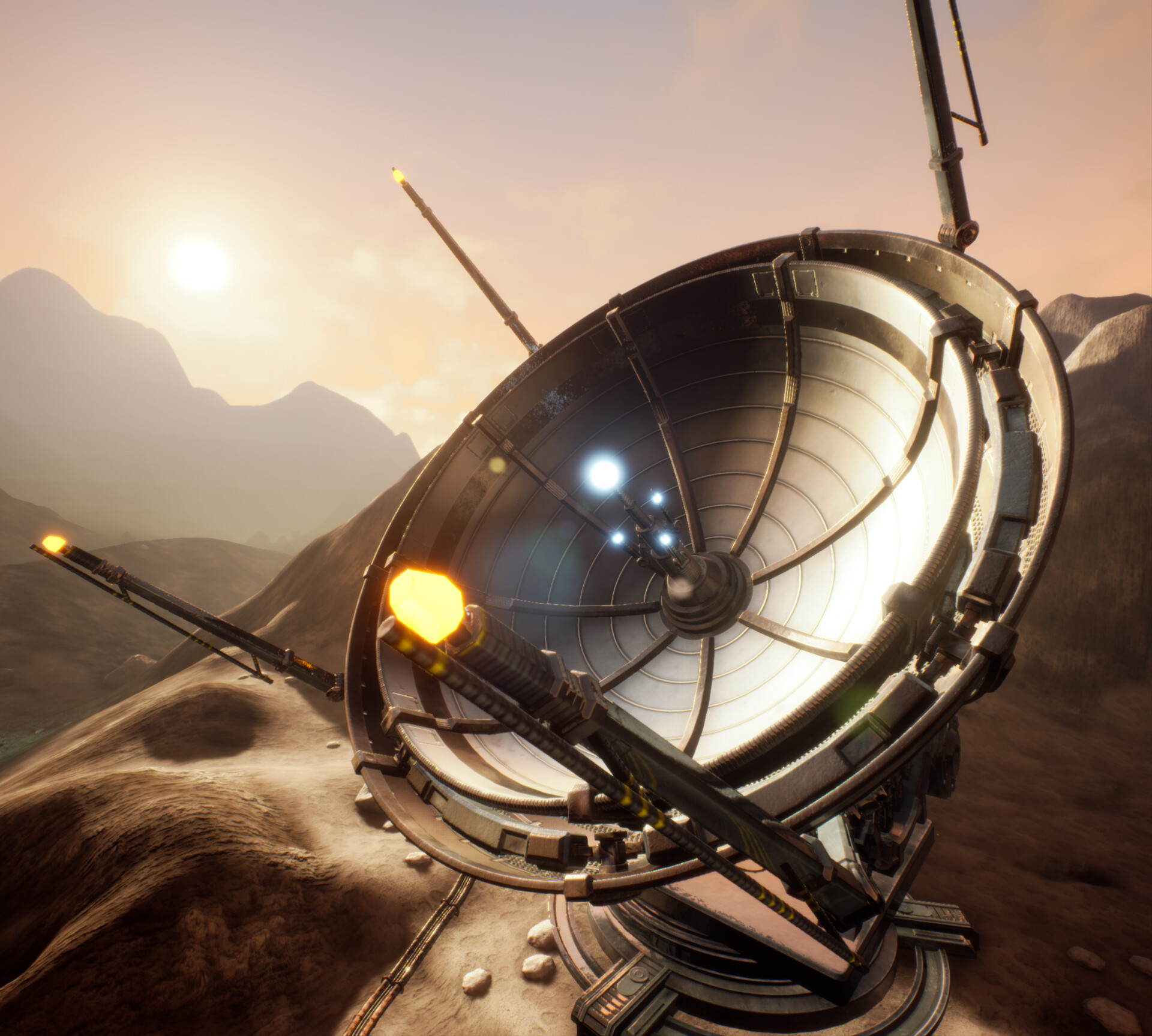The image captures a stylized and ornate satellite dish, likely AI-generated or painted, set on a smooth, rocky terrain with steep, craggy mountains in the background. The terrain around the dish is remarkably smooth, devoid of vegetation and showing no signs of natural weathering, giving it an artificial appearance. The sky overhead is a striking purple and pink hue, suggesting either sunrise or sunset, with the sun visible and casting a bright light. The dish itself is mounted on a solid base station and faces upward at a slight angle towards the sky. Four metallic rods extend outward from various parts of the dish's edge, each tipped with bright yellow or orange lights. The dish's surface is intricate, with significant ribbing and structural details, including visible wiring and multiple lights— a large circle of light on the upper rim and smaller circles below it. Pebbles lie scattered around the base, enhancing the rugged yet smooth appearance of the terrain.